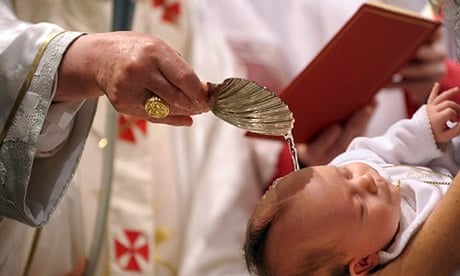The image captures a serene moment of a baby's baptism. The baby, dressed in a lovely white outfit, is held securely in the arm of a parent, with its eyes gently closed, radiating a peaceful aura. Holy water is being delicately poured over the baby's head from a golden, seashell-shaped vessel held by a Catholic priest. The priest is adorned in white, billowing silk robes accented with red crosses and gold etchings on the sleeves. On his finger, a prominent gold ring glistens as he performs the sacred ritual. Nearby, another person's hands—possibly feminine—are visible holding a thick red book, adorned with a red ribbon bookmark, presumably containing the baptismal blessings. This close-up shot focuses on the baby's tranquility and the solemnity of the religious ceremony, emphasizing the significant details that contribute to the sanctity of the moment.